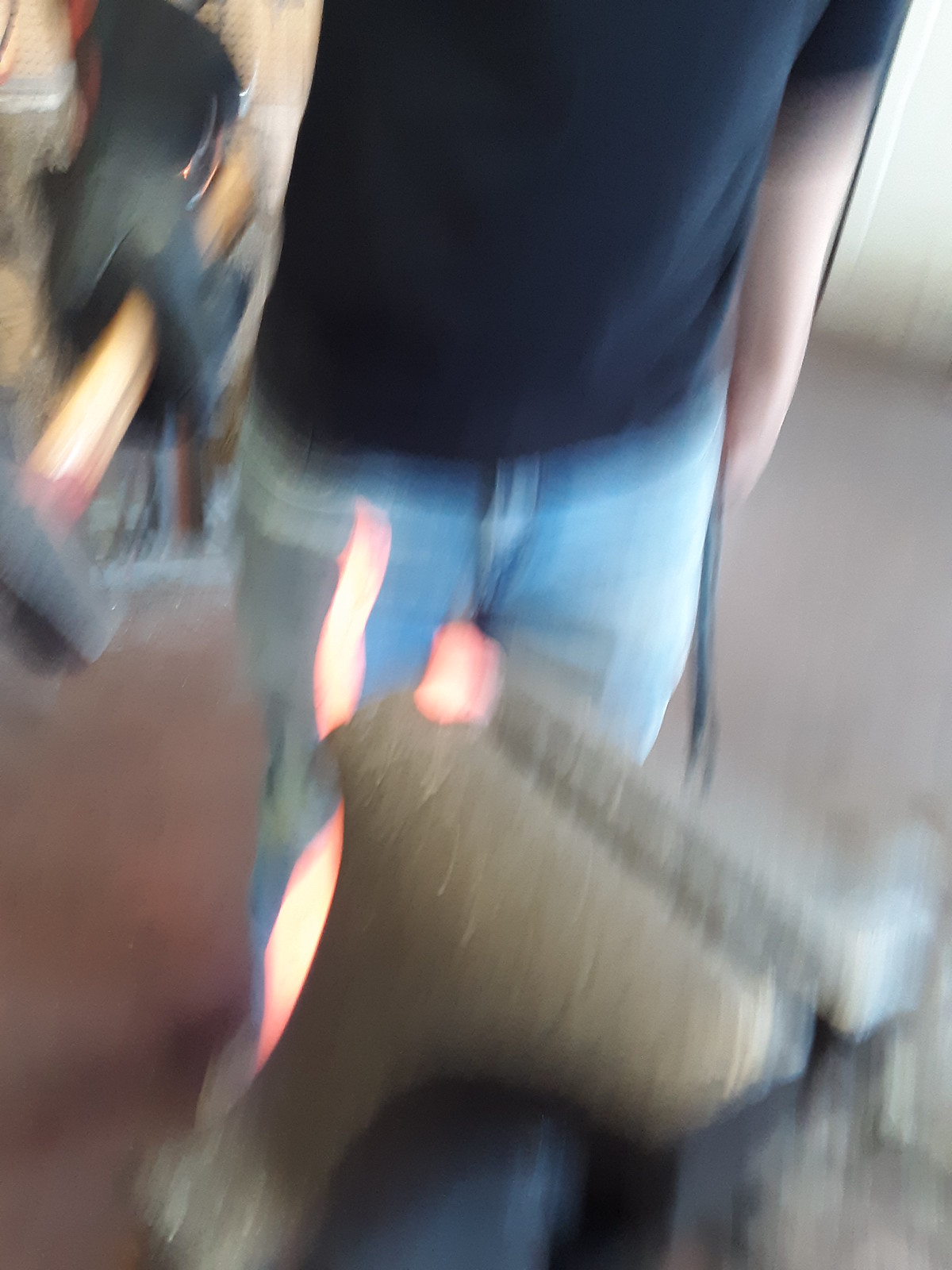In a workshop or possibly a barn-like setting, a man is depicted from the neck down, wearing a black t-shirt and blue jeans. He stands on an industrial, painted red concrete floor. In his gloved right hand, he holds a hefty, long-armed hammer, poised to strike a glowing, red-hot piece of metal clamped securely on a workbench. The large clamps are robust, heavy-duty, and resemble those used in woodworking. A wire can be seen extending from the workbench area, adding to the industrial feel of the scene. The man's left hand hangs by his side, and the metal in the clamps emits a bright reflection on his blue denim jeans. The image provides a glimpse into the intense, hands-on labor involved in metalworking.